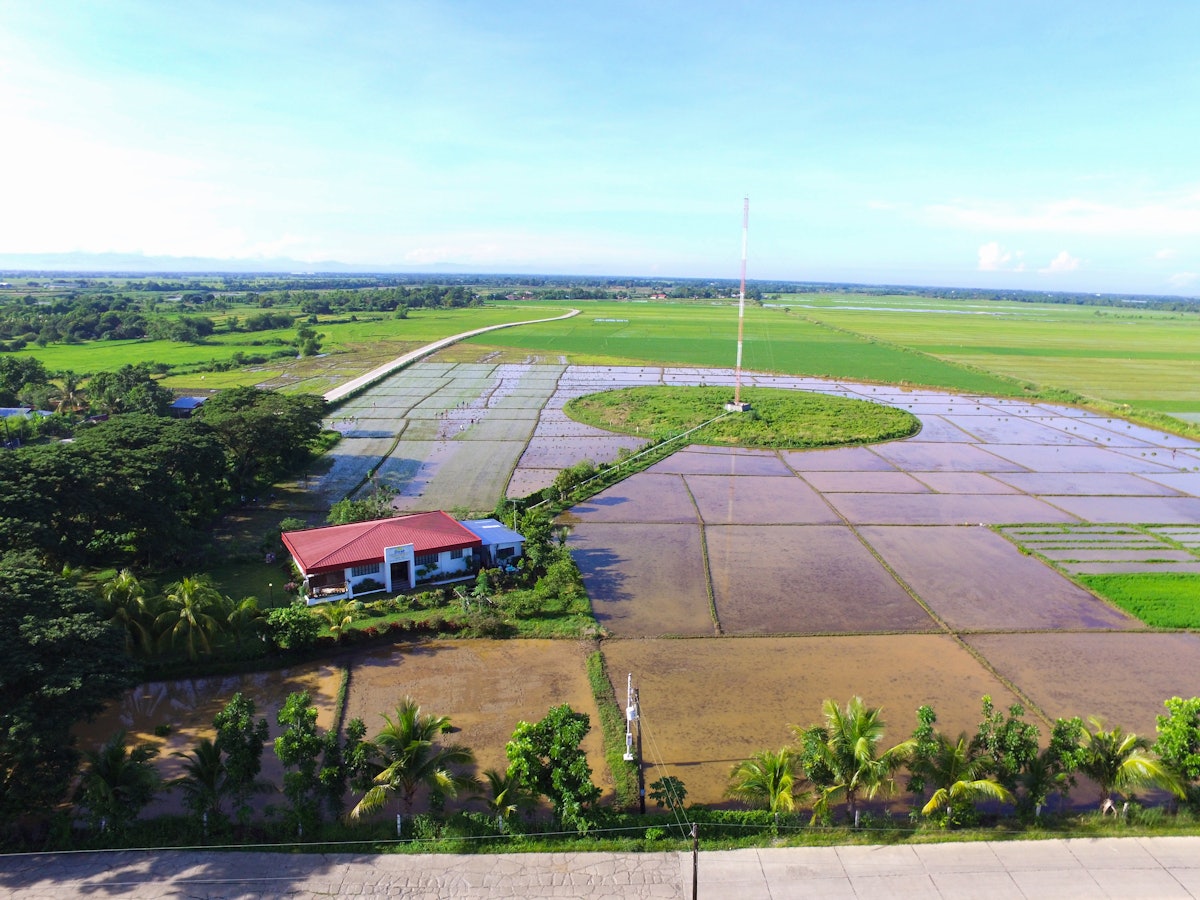The photo captures an expansive, flat agricultural field extending into the horizon, resembling the vast landscapes typical of the Midwest. At the center of the image is a distinctive rectangular building with a red roof and white walls, likely of commercial or residential use, featuring signage above its entrance. A narrow grass strip or pathway leads from this building to a large circular green lawn, distinctively surrounded by a tall red and white pole, possibly a radio tower, supported by tension cables. The area surrounding the building and circular lawn is composed of small brown rectangular plots, suggesting dirt or paved farming plots that might be reminiscent of rice paddies. To the left of the building, a dense cluster of trees provides a contrasting backdrop, with some smaller, palm-like trees in the foreground adding a tropical touch. The sky above is a clear blue with a few light clouds, suggesting a sunny day. In the distance, on the left side of the image, faint mountains can be seen, adding depth to the serene agricultural scene.